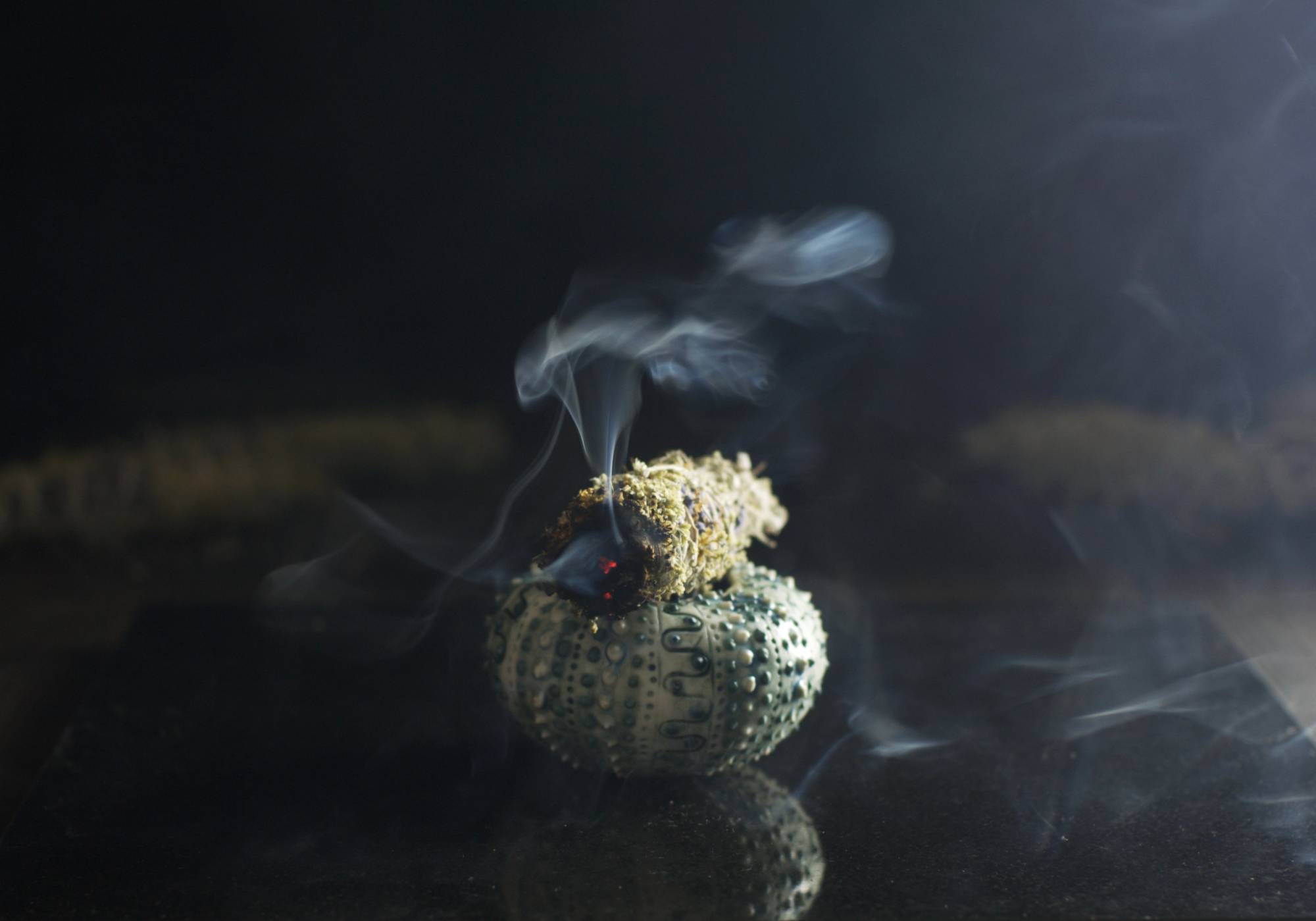The image features a smoldering sage stick centered horizontally just below the middle of the frame. The sage stick, emitting a swirl of white-gray smoke that fills the air around it, sits atop a small, intricately designed, tan-colored object, which resembles a pincushion or a round seashell. This base is adorned with vertical lines comprised of raised beads or push pins, adding texture and detail. The background is predominantly black, adding a stark contrast that highlights the smokey trails. Blurred and indistinct shapes in the background suggest additional objects lying on a table, but their details are obscured by the lighting and smoke.